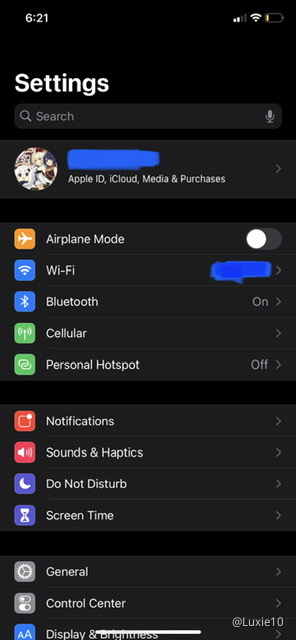A screenshot showcases a phone's settings menu against a completely black background. Located in the upper-left corner, "6:21" is displayed, along with two bars indicating weak internet connectivity and an extremely low battery level, estimated at around 10%, though no exact percentage is shown. 

At the top of the settings menu, a search bar is visible. Just below it, an icon, marked out in blue, indicates access to the user's "Apple ID, iCloud, media, and purchases." Following this, a series of settings options are listed, each accompanied by its respective icon on the left:

- **Airplane Mode**: Turned off.
- **Wi-Fi**: Unavailable or blued out, rendering it unreadable.
- **Bluetooth**: Turned on.
- **Cellular**: Disabled, though it features a clickable option.
- **Personal Hotspot**: Turned off, with a clickable toggle.

The menu continues with additional clickable options:

- **Notifications**
- **Sounds & Haptics**
- **Do Not Disturb**
- **Screen Time**

Following a separating line, the settings options are further categorized:

- **General**
- **Control Center**
- **Display & Brightness**

Each setting label is prominently displayed, but none of the submenus are expanded.